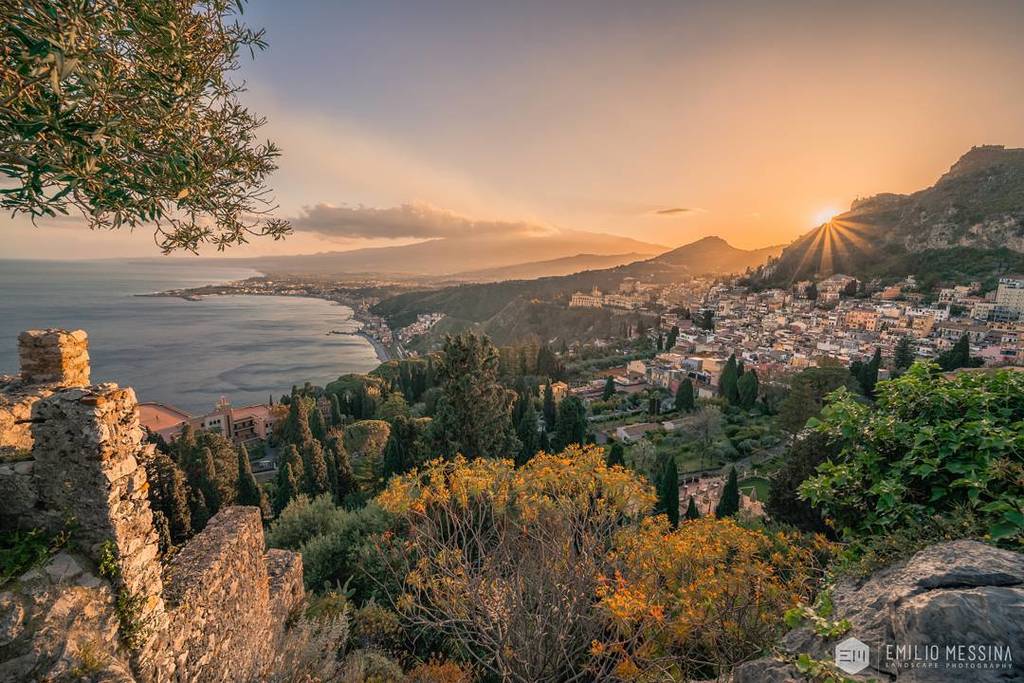This stunning landscape photograph, signed by Emilio Messina in the bottom right corner, elegantly captures a picturesque seaside village in Sicily from an elevated vantage point. The scene is bathed in the warm amber glow of either a rising or setting sun, which peeks over distant mountains, casting radiant sunbeams and creating a striking striation effect in the pale gray sky. At the forefront, a weathered stone wall and an array of native plants, including vertical shrub-like trees, frame the idyllic view. To the left, a tall green tree adds depth and contrast to the composition. The image reveals a bustling hillside village with numerous buildings cascading toward a curved shoreline, where the blue-green sea meets the edge of a cliff. The serene water stretches into the horizon, dotted with additional distant structures. This captivating photograph beautifully encapsulates the rustic charm and natural splendor of Sicily’s coastal landscape.